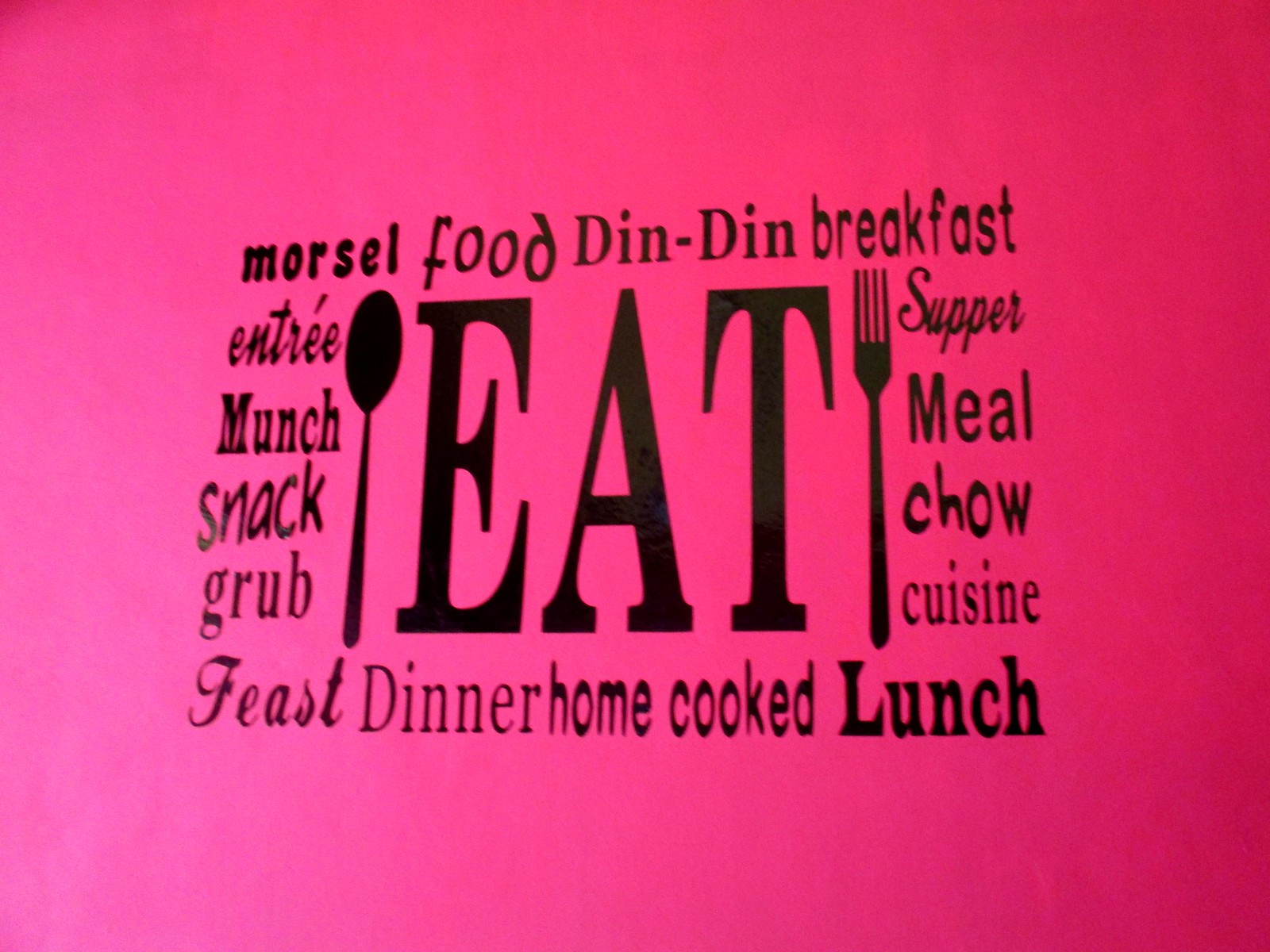The image is a vibrant advertisement for a restaurant or menu, predominantly featuring a bright pink to reddish gradient background that transitions from brighter on the left to darker on the right. Centered in bold, black letters is the word "EAT," with a black spoon to the left of the "E" and a black fork to the right of the "T." Surrounding "EAT" are various words related to food, each in a unique font. Starting from the top left, the words "MORSEL," "ENTREE," "MUNCH," "SNACK," "GRUB," and "FEAST" cascade vertically. At the top of the image, the words "MORSEL," "FOOD," "DIN DIN," and "BREAKFAST" stretch horizontally across. To the right of the fork, from top to bottom, are "BREAKFAST," "SUPPER," "MEAL," "CHOW," "CUISINE," and "LUNCH." Beneath "EAT," words such as "DINNER," "HOME," "COOKED," and "FEAST" are prominently displayed. The diversity of fonts ranges from rounded and cartoonish to Times New Roman and cursive, adding visual interest to the advertisement.